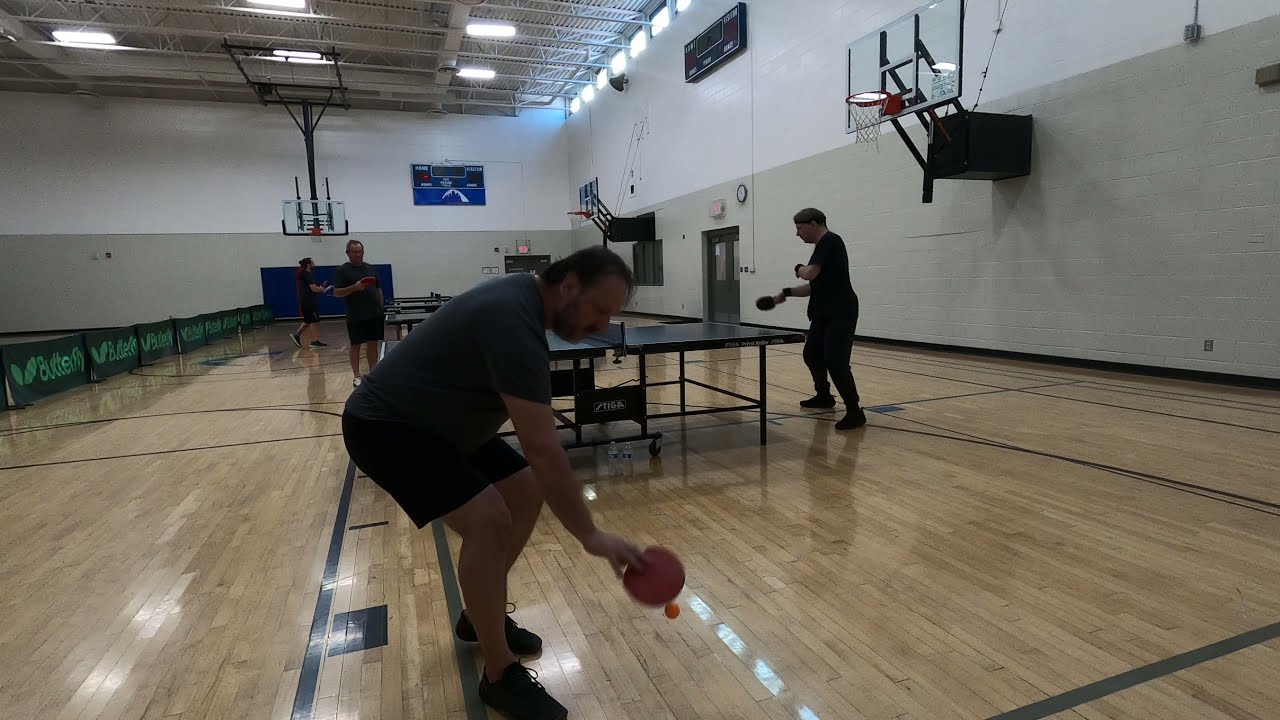The photograph captures a lively scene inside a high school gymnasium devoted to a ping pong activity. Dominating the foreground, a man is centered, dressed in black tennis shoes, black shorts, and a dark gray t-shirt. He stands with bent knees, focusing intently on bouncing a small red ball with a paddle. His short brown hair and possible facial hair are slightly blurred. To his rear, another ping pong player in an all-black short-sleeve outfit is mid-action, poised with his right hand extended to hit the ball. Further back, another individual stands at a ping pong table, engrossed in something in his hands, while a woman nearby participates in another ongoing game. The gym’s ambiance is highlighted by white upper walls and gray lower sections, with multiple fluorescent lights suspended from the ceiling. The hardwood floor is marked with traditional black basketball lines, complementing the visual markers of basketball rims and a scoreboard in the background. Overall, the image captures a dynamic environment where numerous participants are either preparing for or actively engaged in ping pong gameplay.